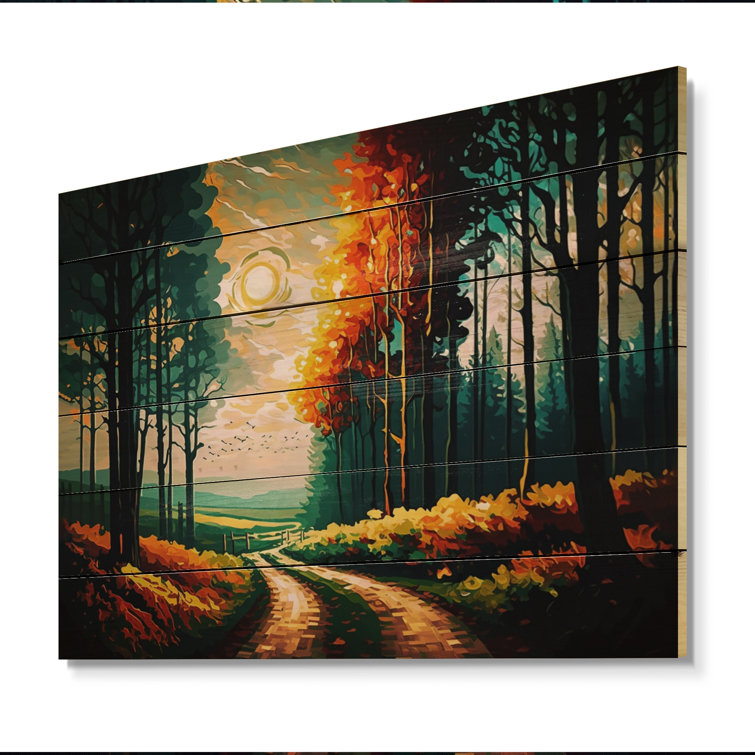This captivating painting, displayed against a clean, white background, features a serene country dirt road winding through a vividly colored autumn landscape. The sky, painted in light beige, cream, and hints of green, showcases a setting sun that bathes the scene in warm light. In the distance, gently rolling green mountains provide a tranquil backdrop, with farmland fields delineated by clusters of trees.

The foliage reflects the transition of seasons with a mix of green, yellow, and orange leaves, creating a tapestry of vibrant fall colors. The painting includes a variety of trees, including deciduous ones and some pine trees visible in the far-right background. In the foreground, the road appears divided by a green grass strip, and both the road and surrounding grasses exhibit hues of orange and green. Despite some suggestions of lines resembling power lines, these appear to be artifacts from the frame rather than part of the artwork. The overall composition of trees, distant fields, and the winding trail under a softly setting sun evokes a peaceful, rustic charm.